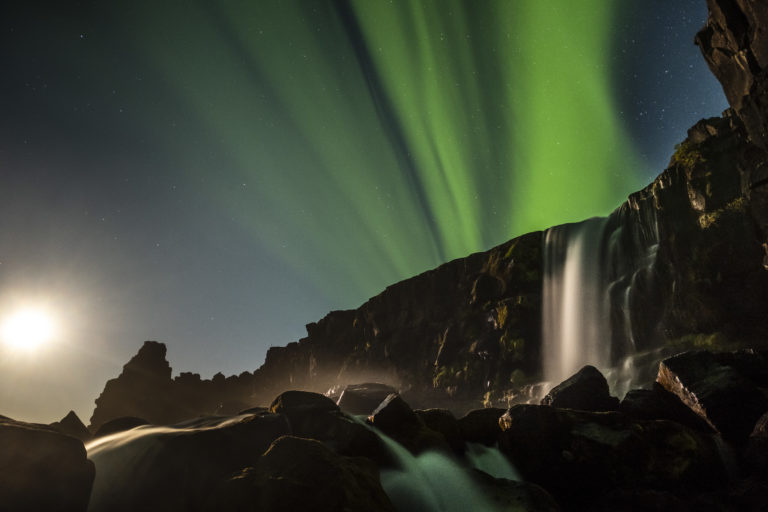In this detailed outdoor image, a scene unfolds at either dawn or dusk, with the sun positioned on the lower left side, casting a silvery white light that touches the rocky terrain beneath. Dominating the sky above is a dark blue expanse adorned with stars, interspersed with vibrant green streaks resembling the Northern Lights, shooting upwards from the middle of the picture. In the foreground, you can see rugged, orange and yellow rocks, with water running across and cascading down them in two distinct spots—one towards the bottom left and another towards the middle bottom. The rocky formations grow larger towards the right, forming imposing cliffs or mountains. From these towering rocks on the right side, a striking waterfall spills over, its white, foamy waters descending gracefully over the textured surfaces, creating a mesmerizing interplay between the elements.